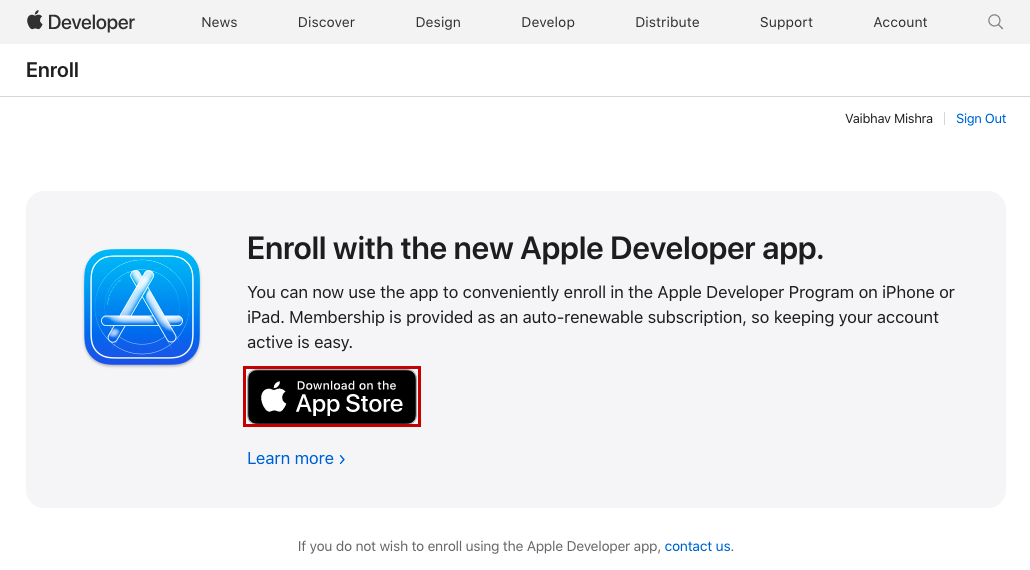This image is a screen capture taken from a desktop computer. The screen has a white background and features a horizontal bar at the top in a very pastel shade of grey. On the far left of this bar is the iconic Apple logo, characterized by the bite taken out of it. Next to the logo, "Developer" is written in black. Moving right across the bar, the following headings are listed in sequence: News, Discover, Design, Develop, Distribute, Support, and Account.

In the main body of the screen, there is a prominent header written in bold black text: "Enroll with the new Apple Developer app." Directly below this header, a subtext in black reads, "You can now use the app to conveniently enroll in the Apple Developer Program on iPhone or iPad." To the left of this text, there is a logo consisting of a capital letter "A" on a blue square background with rounded corners.